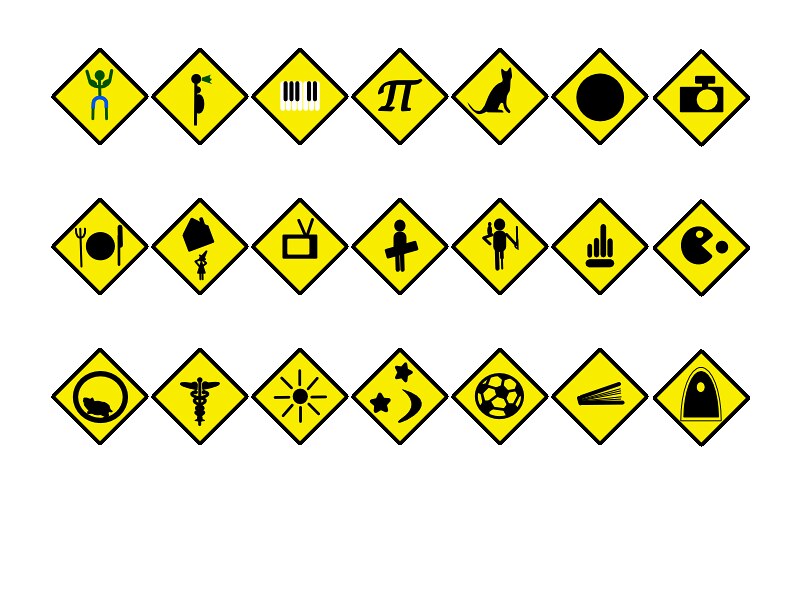The image features a collection of various symbols, each enclosed within a yellow diamond-shaped square. The symbols are organized into three rows, with each row containing seven distinct symbols. Here's a detailed description of each row and its symbols:

**First Row:**
1. A person holding their arms up.
2. A side view of a person who appears to be talking.
3. Piano keys.
4. A symbol that looks like a number or writing character.
5. A cat.
6. A black circle.
7. A camera.

**Second Row:**
1. A fork, plate, and knife.
2. A house situated above a person.
3. A TV.
4. A person holding a board.
5. Another person with what seems to be a bird or pet on their shoulder.
6. A graph with lines of varying lengths.
7. A Pac-Man-like symbol about to eat some food.

**Third Row:**
1. A hamster in a wheel.
2. A lifeline or medical symbol.
3. The Sun.
4. Two stars and a moon.
5. A soccer ball.
6. A stapler.
7. An archway with a yellow dot in the center.

This detailed arrangement of diverse symbols within a consistent background provides a rich and intriguing visual experience.